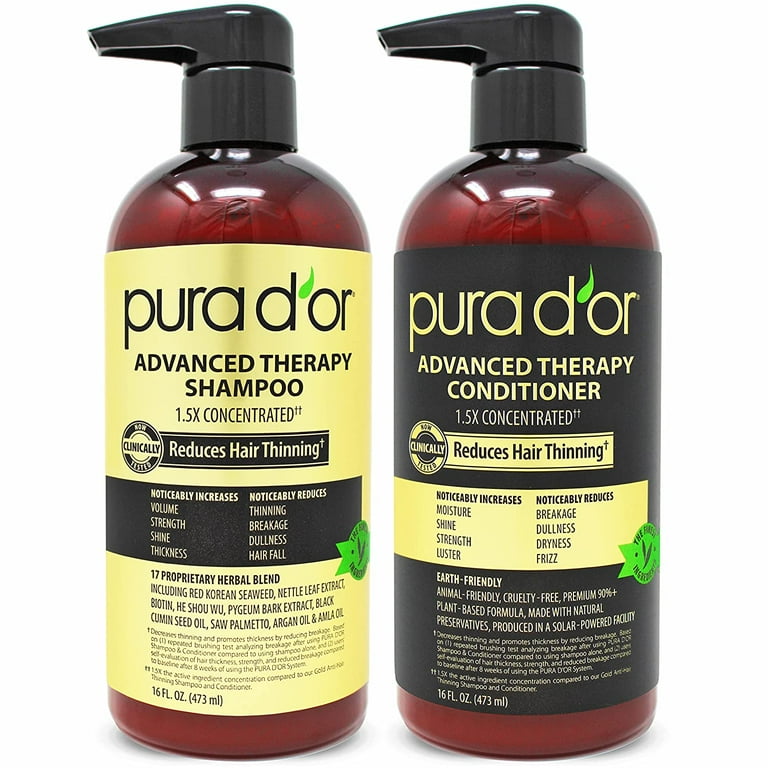The close-up, professionally-captured image features two brown glass bottles of hair products from the brand Purador, set against a sterile white background. Each with a black, duckbill cap, the bottles are labeled similarly in detailed golden text with distinguishing features. The shampoo bottle on the left sports a yellow label and reads "PuraD'or Advanced Therapy Shampoo, 1.5 times concentrated," highlighting its clinically-tested ability to reduce hair thinning while enhancing volume, strength, shine, and thickness through a blend of 17 herbal extracts. The conditioner bottle on the right mirrors these properties with a black label featuring yellow text, and it focuses on combating hair thinning and breakage. Both products, totaling 16 fluid ounces (473 milliliters) each, also boast ingredients such as seaweed, bark extracts, and seed oils aimed at replenishing hair growth.